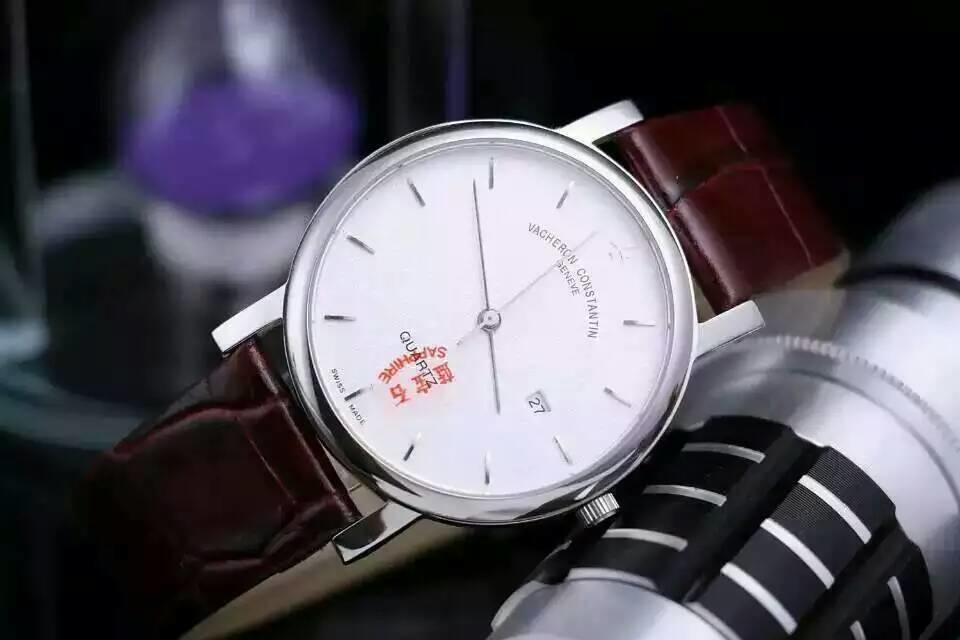This is a detailed description of a distinctive Swiss-made watch. The watch features a minimalist design characterized by a gray dial set against a white background. Instead of traditional Roman numerals or Arabic numbers, the watch uses 12 simple lines to mark each hour. Notably, there are no dots to indicate the minutes, but there is a system in place with lines every 15 minutes for clearer time distinction. 

The watch includes a date area and proudly bears the inscription "Swiss Made," a hallmark of its origin. The time is displayed with three hands – hour, minute, and second – each elegantly designed for precision. The hands stand out against the background in black, ensuring high readability.

The timepiece is complemented by luxurious red-burgundy leather straps, adding a touch of sophistication and comfort. The watch also carries a notable red stamp that reads "Course Order," which adds an element of intrigue, as it is not commonly seen. The minute and hour markers are crafted from small, refined silver metal pieces, contributing to the watch's overall sleek and modern aesthetic.